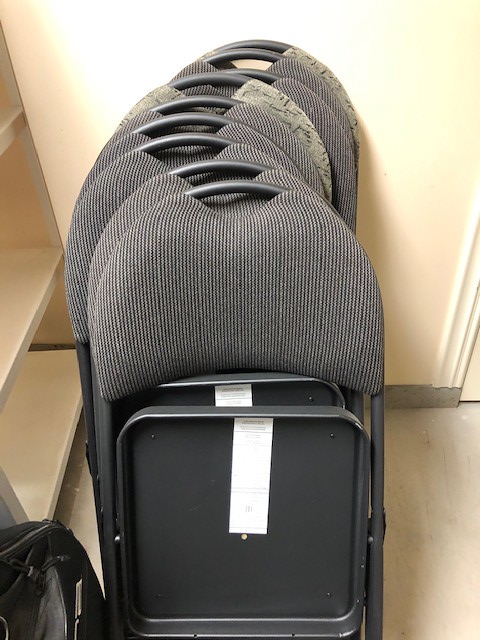This photograph features a set of nine or ten dark gray folding chairs, stacked haphazardly in a somewhat disorganized line, leaning against a cream-colored wall with white trim in a small closet. The room has pinkish-gray flooring and some shelves that highlight its tight space. Two of the chairs stand out with a slightly different green-gray pattern, contrasting with the otherwise uniform gray chairs. The baseboard appears to be a shade of gray, adding to the detailed elements in this confined storage area.